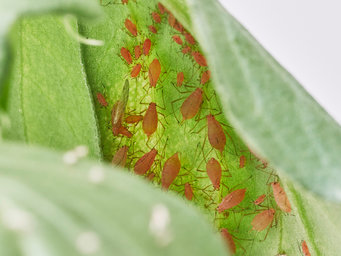This image is an extreme close-up of a leaf, likely taken indoors or in a laboratory setting, given the controlled white background observed on the right-hand side. The leaf itself, displayed in intricate detail, reveals its green parts and fibrous veins. Upon closer inspection, one can see a variety of small, light brown to orange insects dispersed across the leaf. The insects vary in size, with larger ones predominantly positioned on the bottom right, moving towards the top left, and smaller ones clustered in the top left. The foreground on the lower left features an out-of-focus portion of another leaf, adding depth to the image. The background in the upper right corner is a vacant white space, possibly indicative of an artificial backdrop. The collective appearance of the insects and the precision of the close-up suggest an infestation on the leaf, highlighting the pests with detailed clarity, including discernible legs and occasional wing-like structures.